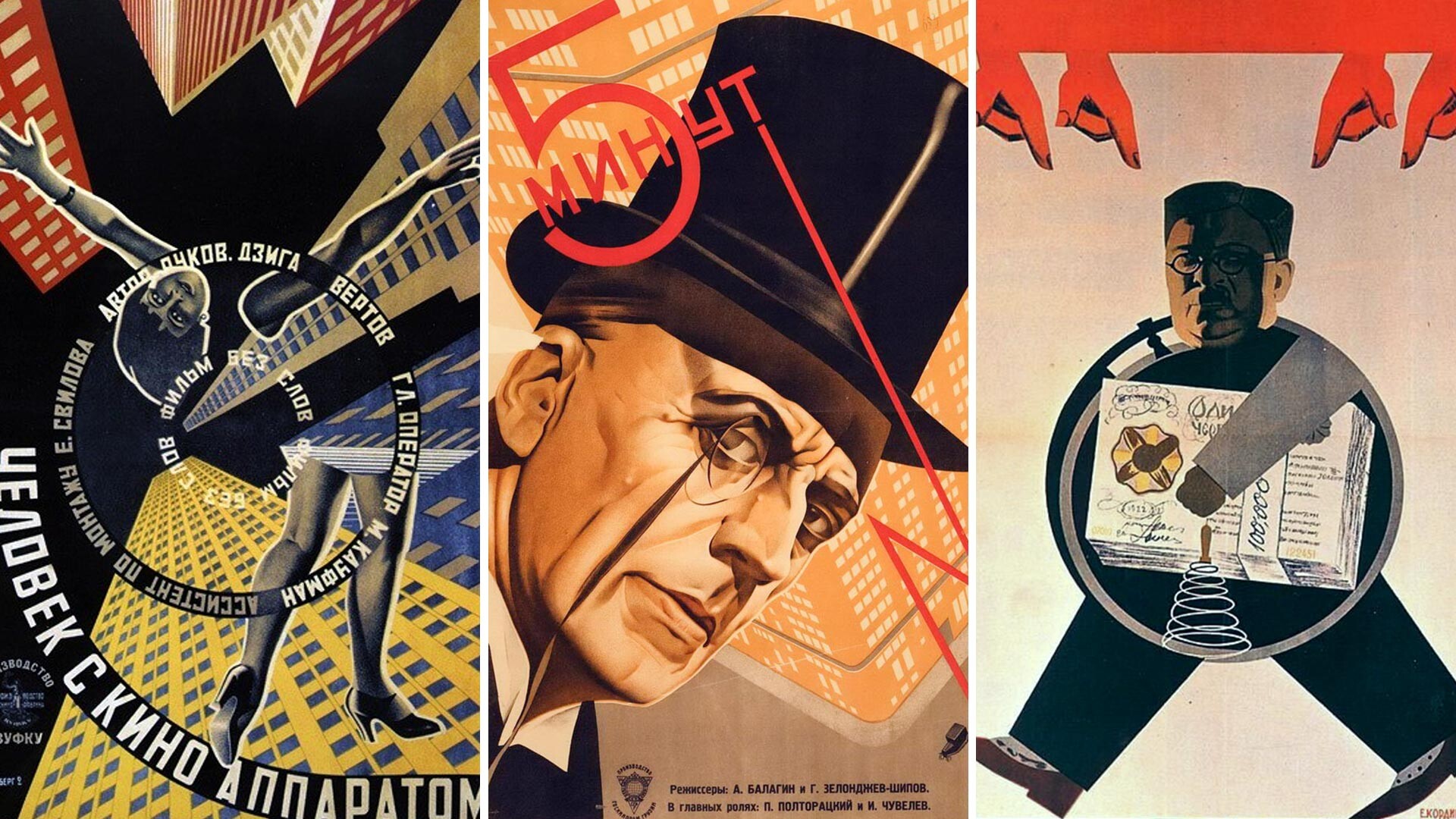The image comprises three distinct pictures arranged side by side. 

The left picture features a high-contrast scene with a black background, intended to depict the night sky. City buildings are presented upside down in various colors, including red, yellow, and blue. Dominating the scene is a woman with black hosiery and high heels, her arms outstretched and her head tilted back, creating an impression that the buildings rest atop her. The image is encircled by what appears to be Russian text, arranged in a hypnotic circular pattern.

The central picture showcases a man wearing a shiny black top hat and small, round glasses. He appears to be gazing directly at the viewer with a calm demeanor. A large red number '5' is prominently displayed over his chest, and the letters 'MNHYT' are written beside it, with the 'T' extending into a downward arrow. In the backdrop, a high-rise building can be faintly seen, and illegible black text forms the base of the composition.

The right picture is bordered in red with four hands, each pointing downward with extended index fingers, two on the left and two on the right. Central to this image is a man with black hair, glasses, pants, and shirt, encapsulated within a gray circle. His left arm is notably gray, and he holds numerous white cards covered in writing. His figure is boxy, encompassing a round body with squared arms and legs, and he too seems to be looking directly at the observer.